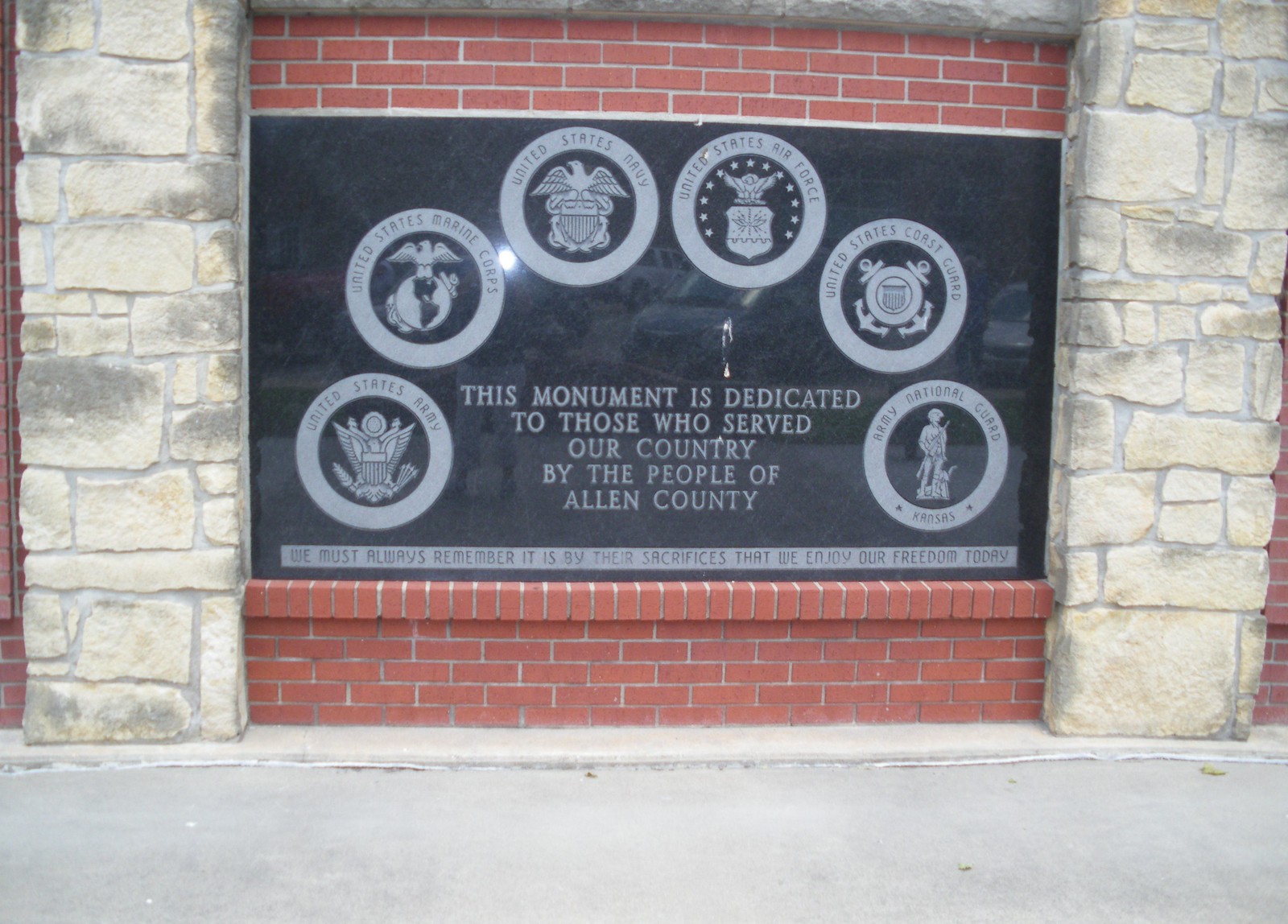The photograph captures a monument featuring two cream-colored stone pillars framing a red brick wall with gray grout. Centered on the wall is a black plaque displaying six gray-circled logos, each representing different branches of the United States military. From left to right and bottom to top, the logos are for the United States Army, Marine Corps, Navy, Air Force, Coast Guard, and Army National Guard from Kansas. The Army logo depicts a bird with a crest, while the Marine Corps logo showcases a globe with an eagle. The Navy and Air Force logos feature crests with eagles and stars. The Coast Guard logo has anchors at the top and bottom, and the Army National Guard logo depicts a historic soldier holding what appears to be a rifle or flag. Framing these logos in a semicircle, the plaque reads: "This monument is dedicated to those who served our country by the people of Allen County." Below this dedication, another inscription states: "We must always remember it is by their sacrifices that we enjoy our freedom today." The image is slightly cropped, revealing part of the sidewalk at the bottom.